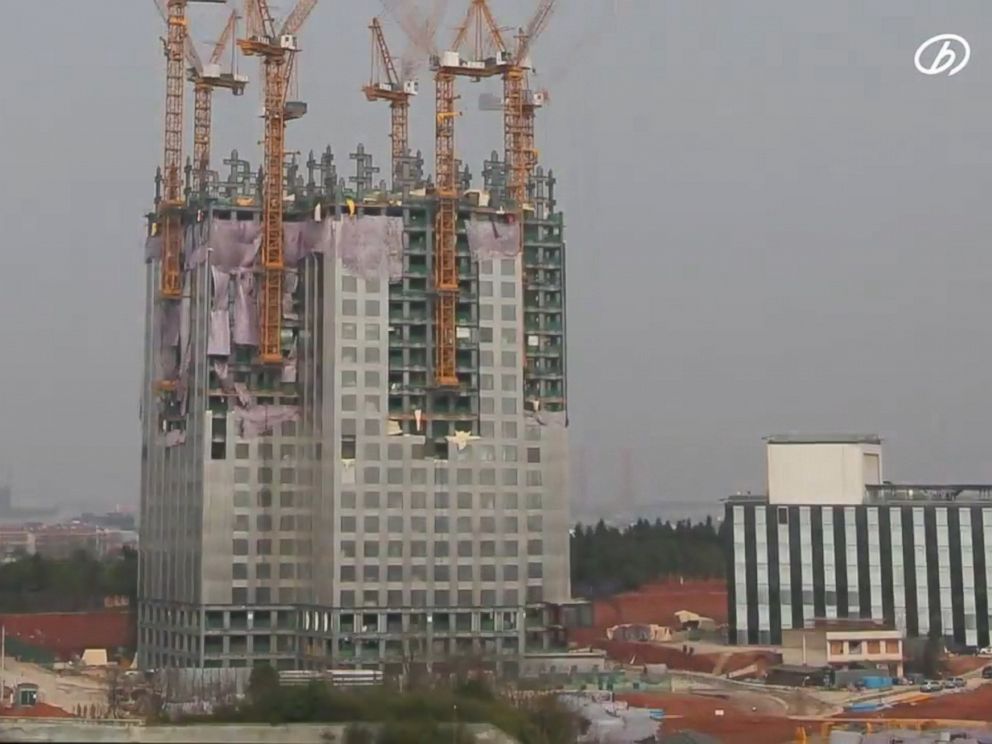The image depicts a high-rise building under construction, possibly in China, that appears to be around 20 to 30 stories tall. The structure, predominantly gray and blocky, features a concrete base with a steel framework extending upwards. The building is wrapped in scaffolding and other construction materials, particularly around the windows, indicating ongoing work. A total of six cranes are strategically positioned around the building, aiding in the lifting of materials. The top portion of the building is unfinished, with yellow structures visible for construction workers to navigate. At the base, there are red-hued low-rise buildings and a zebra-striped building to the right. The weather is overcast and hazy, with a gray sky tinged faintly blue. In the distance, dark evergreen trees are noticeable, and the ground appears dry and sand-like. The emerging skyscraper stands as the tallest structure in the vicinity.